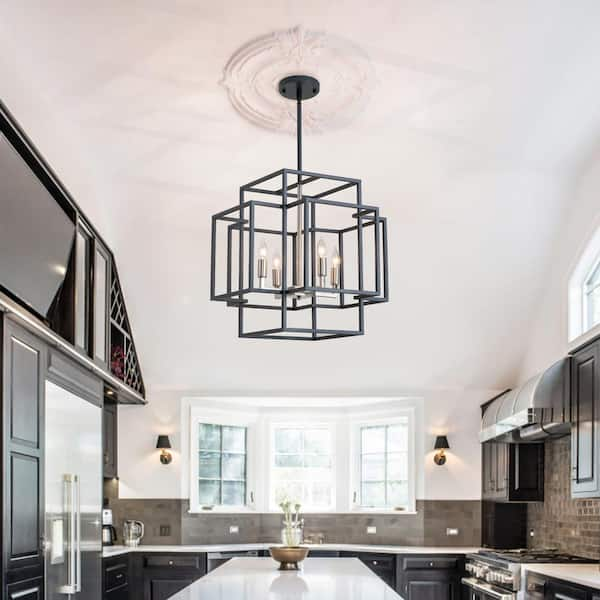The image captures the interior of a sophisticated, modern kitchen bathed in an airy, white ambiance, contrasted by sleek, dark black cabinetry and appliances. Dominating the scene is a striking chandelier made up of overlapping geometric metal rectangles arranged symmetrically, with faux candle-like lights nestled within. The chandelier, rendered in a brushed black metal, is mounted to the ceiling, which features an ornate sculptural plaster element, adding a touch of elegance. The kitchen’s centerpiece is a large island topped with white quartz or marble, aligning with the three inset windows that flood the space with natural light. Below the windows, a sink is flanked by two black and gold sconces, complementing the modern aesthetic. On the right, a stainless steel stove with a vent hood stands against a backdrop of smooth, shiny gray brick-like stone, while additional pantry storage and a refrigerator occupy the left side. This stylish kitchen, outfitted with necessary appliances and accentuated by high-quality finishes, epitomizes the blend of functionality and contemporary design, akin to an impressive setup you'd find in an architectural digest magazine.